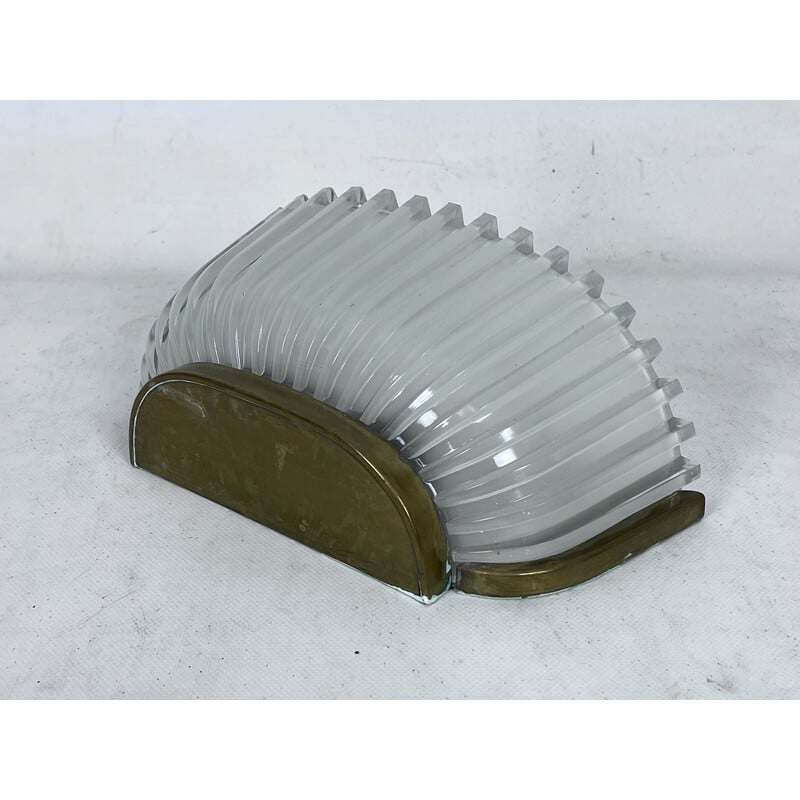The image showcases a vintage-style light fixture that appears to date back to the 1950s or earlier. It features a see-through glass dome, reminiscent of a seashell or slinky, stretched across from the bottom right corner to the top left corner. The base of the lamp is a greenish, olive-colored or potentially gold hue. The glossy and shiny plastic of the fixture catches light, creating a striking contrast against the gray and white smudged background. Positioned centrally, the light fixture stands out prominently, offering a nostalgic yet artistic ambiance.